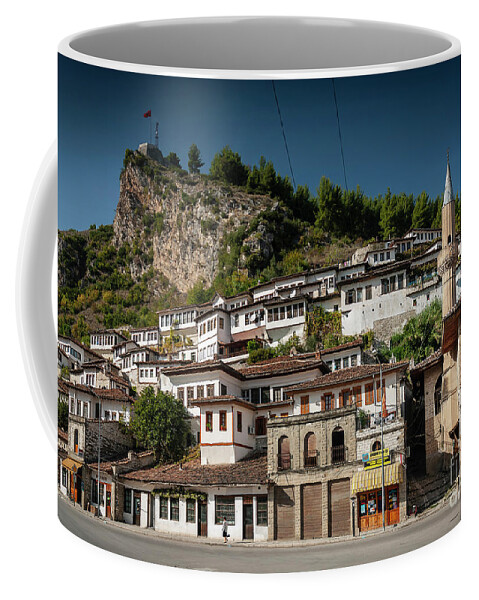This image depicts a coffee mug that features an elaborate countryside village scene printed on its surface. The main part of the mug, which appears to be a light green color, showcases a picturesque image dominated by a series of houses scaling up a hill or mountain. The houses are mostly white with dark brown and reddish roofs, creating a charming and rustic feel. Behind the houses, the hill is adorned with green trees, possibly pines, adding depth and natural beauty to the scene. At the top of the hill, there is a small building crowned with a red flag, hinting at either a fort or some other significant structure. Above the hill and trees, the sky is a striking blue, providing a vibrant backdrop to the village scene. The mug’s left side reveals part of a white or cream-colored handle, forming a contrast with the light green background. The image is detailed down to the white rim of the mug and the visible part of its interior which appears to be white or cream. The background of the entire image is a clean, stark white, ensuring all attention is focused on the detailed and picturesque scene printed on the mug.